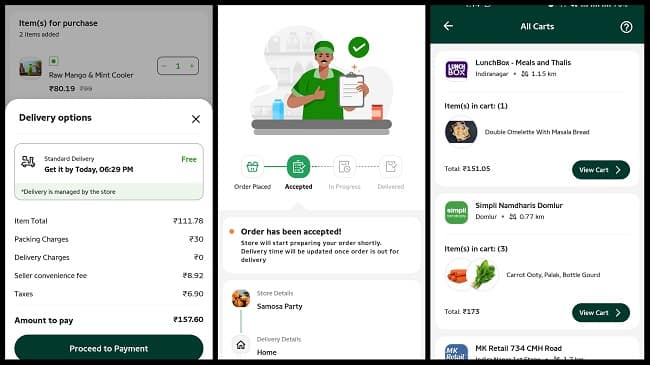The photograph depicts a detailed interface of an online grocery shopping experience. Central to the image is a man, possibly a store clerk or doctor, in a green shirt and hat, seated behind a counter, holding a clipboard. This setting appears to be within a grocery store.

The main screen showcases various order details:

- **Product Selection**: 
  - "Raw Mango and Mint Cooler" is selected, with a promising delivery option stating "Get it today for free."
  - The total item cost, obscured by a blur, is shown as 111.78 in an unidentified currency.
  - Additional charges are listed: 
    - **Packing Charges**: 30
    - **Delivery Charges**: 0
    - **Convenience Fee**: 8.92
    - **Taxes**: 6.90
  - The final amount to be paid is 157.60.

- **Checkout Process**: 
  -"Proceed to Payment" option illustrated on a blue-and-white capsule button.
  - Sequential order statuses tracked: "Order Placed," "Accepted" (highlighted), "In Progress," and "Delivered." A note indicates, "Your order's been accepted. The grocery store will start preparing your order shortly. Delivery time will be updated once the order's out for delivery."

Below this, more information is provided including options such as "Samosa Party" and "Home Delivery." To the right, an additional section lists more categories such as "All Carts," "Lunchbox," and "Meals."

-An itemized rundown:
  - "Items in Cart: 1"
  - Menu item: "Double Omelet with Masala Bread" for a total of 151.05.

At the bottom, there is another entry for a business possibly named "Simply Nandar's Domler," listing items like carrots and celery with a total of 173 and an option to "View Cart."

No discernible branding or logos are visible throughout the image, making it a generic interface for a grocery store delivery system.